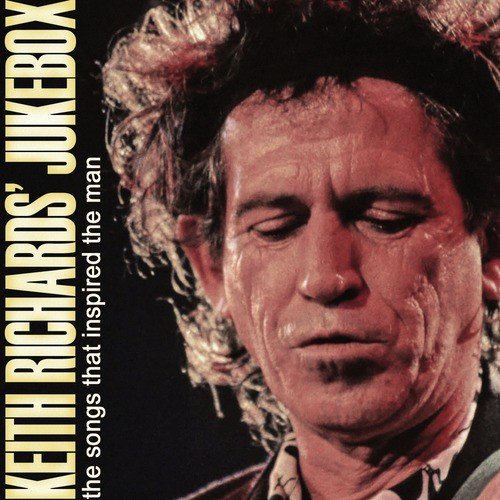The image depicts a middle-aged, wrinkled Caucasian man with short, messy, and rough black hair, appearing to look downward with lips slightly pursed, suggesting a contemplative or focused demeanor. He is dressed in a shirt with a black-and-white pattern, though details of the shirt are indistinct. The background is pitch black, contributing to the emphasis on his face and expression. To the left of the man, text in a golden yellow font reads "Keith Richards Jukebox" vertically, and in white, it states "The Songs That Inspired the Man." The overall color scheme includes black, white, shades of brown, and hints of gold, with a small blue and brown object visible at the bottom right, possibly a strap from a musical instrument. The image has a feeling of introspection, possibly suggesting an album cover.